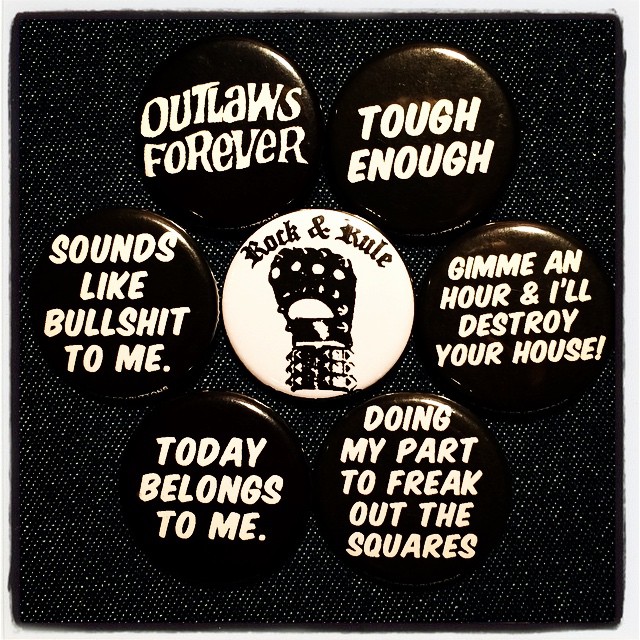This detailed print-style image focuses on a collection of buttons artfully arranged on a black panel. The background is a subtle gray, accentuating the central square graphic. Surrounding a prominent white button with a graphic of a clenched, spiked-bracelet fist, six black buttons with white text form a circle. Reading clockwise, the buttons display the phrases: "Outlaws Forever," "Tough Enough," "Give Me An Hour And I'll Destroy Your House," "Doing My Part To Freak Out The Squares," "Today Belongs To Me," and "Sounds Like Bullshit To Me." The central white button features the bold text "Rock N. Rule." The buttons, featuring a palette of black, white, and off-white, are meticulously centered in the image, suggesting a deliberate and organized collection.